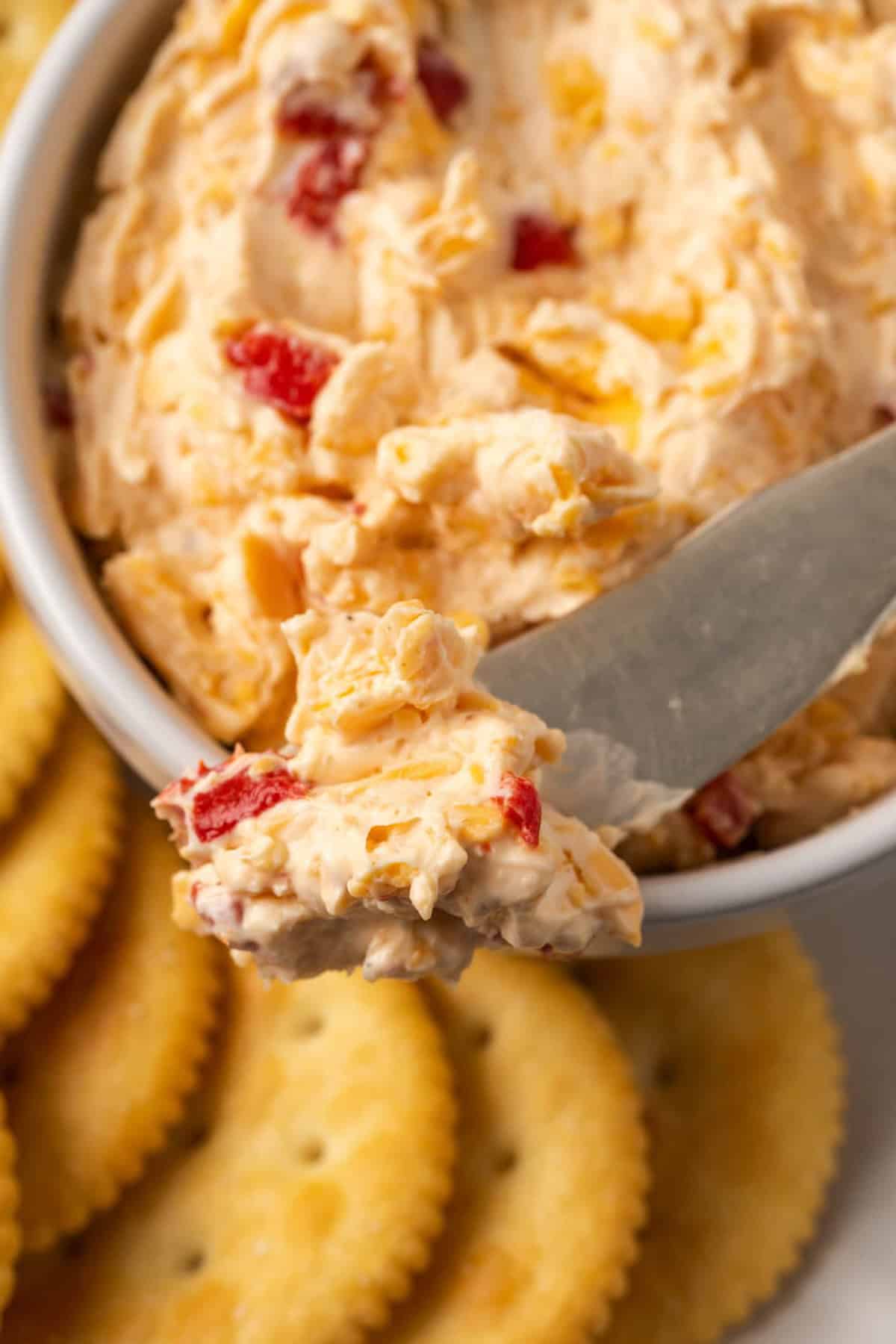This close-up image vividly captures a scene of homemade pimento cheese elegantly presented in a small white porcelain dish. The creamy, textured pimento cheese, speckled with bits of red pepper and various spices, radiates a homemade charm. A butter knife, poised with a generous scoop of the pimento cheese, is positioned prominently, offering a detailed look at the spread's appetizing appearance. Surrounding the dish are golden Ritz crackers, invitingly arranged to enhance the experience of enjoying the cheese spread. The contrast between the cream-colored dish and the golden hue of the crackers adds a vibrant touch to the visually appealing composition, making the entire setup look quite delectable. While the porcelain dish and pimento cheese are sharply focused, the surrounding crackers are slightly blurred, drawing attention to the richness of the pimento cheese.